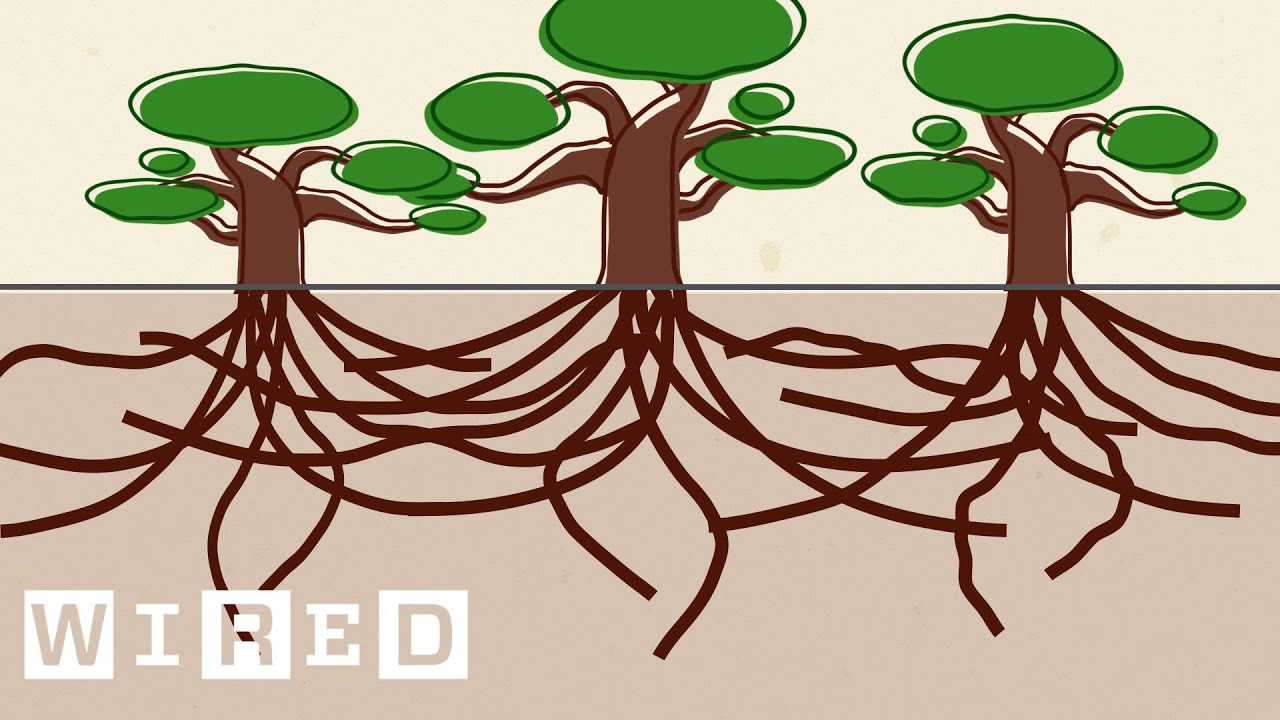This poster features a whimsical, child-like drawing of three trees with brown trunks and clusters of green, circular leaves. The upper half of the poster has a whitish-cream background, while the lower half transitions to a light pink or tan shade. A gray line divides the two sections horizontally. Below this line, thick, wavy brown lines represent the tree roots, crisscrossing and intertwining across the pink-tan area. In the bottom left corner, the text "W-I-R-E-D" is displayed in white against a pink background, suggesting the title or theme of the artwork. The overall composition, with its simple shapes and playful style, indicates that it was likely created by a child, or in a child-like manner, rather than by a professional artist. The colors used include various shades of brown, green, white, pink, and tan.